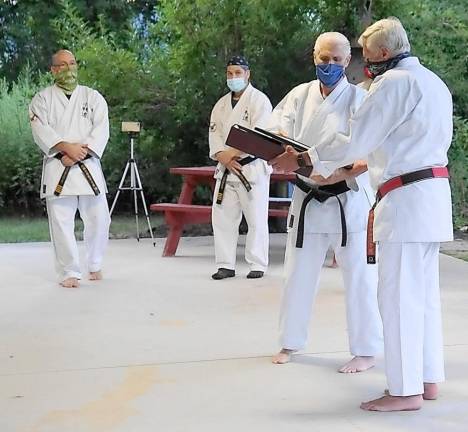The image depicts an outdoor martial arts class, likely a Taekwondo demonstration or test, taking place on a large concrete court. The participants, a group of older men ranging from their 40s to 70s, are all dressed in traditional white martial arts uniforms and are practicing social distancing while wearing masks, indicative of a pandemic-era setting. Among them, three men are wearing black belts—two with gold or mustard yellow embroidery, and the third features a red stripe. Another man sports a red belt. Most of the participants are barefoot, except for one who is wearing black shoes and a bandana. The background reveals lush green trees, a red picnic table, and a setup tripod with a phone, suggesting that the event might be recorded. A man with a blue mask and another with a surgical mask are holding and examining wooden boards, likely preparing for a board breaking demonstration. The sun shines brightly, adding a subtle glow to the scene.